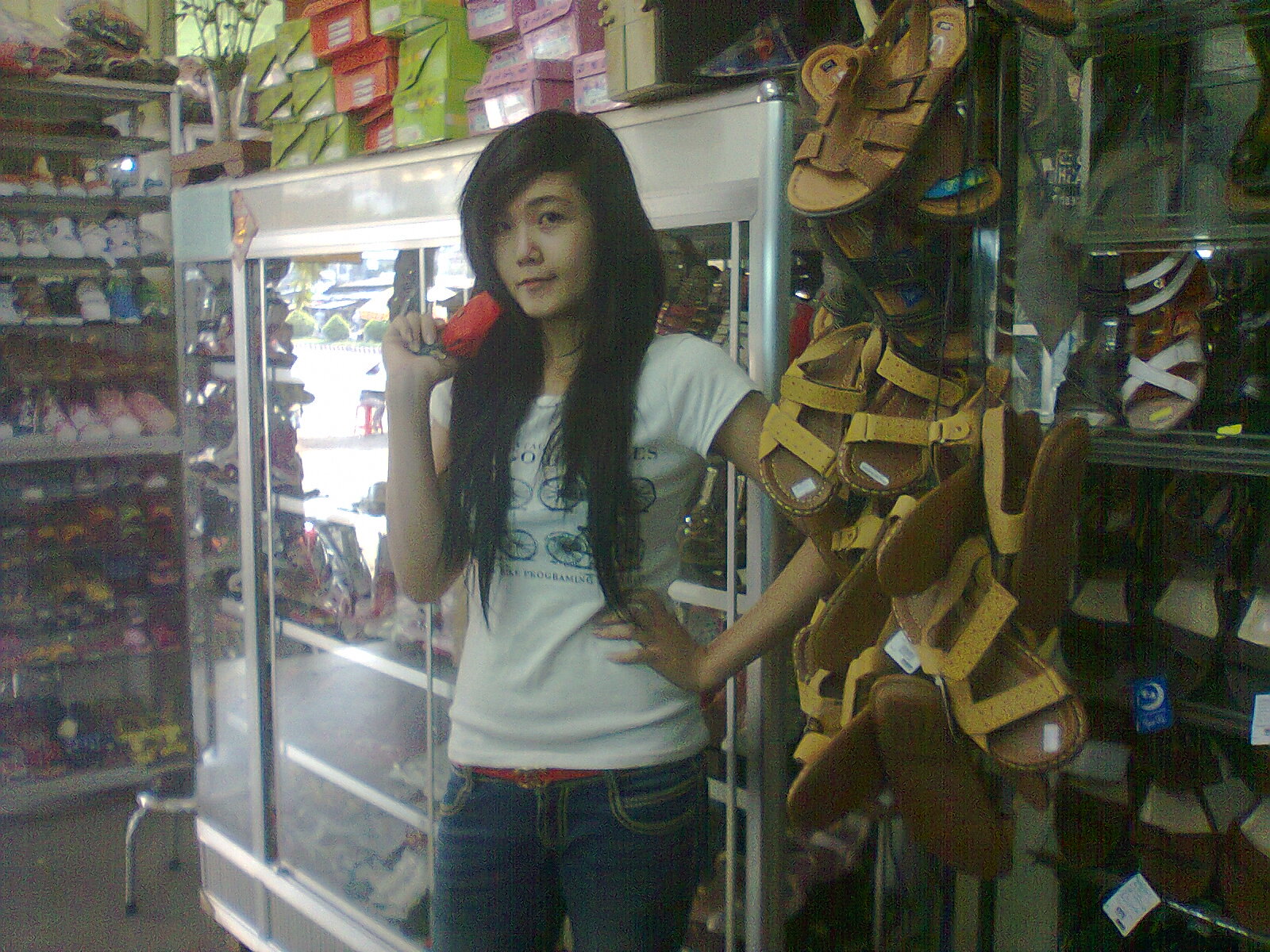In the image, a woman with long, straight black hair is posing inside a store, likely a shoe store. She stands in the center of the photograph, wearing dark denim jeans, a brown belt, and a white t-shirt featuring a green design, possibly bicycles, although her hair partially obscures it. She holds a small red object, possibly a coin purse, close to her face with her right hand, while her left hand rests confidently on her hip.

The store's layout frames her: to her left, there is a prominent wall of neatly arranged shoes in various colors, including pink, blue, and yellow pairs. Beside this, nearer the center, a glass display case catches sunlight, rendering its contents indistinguishable, but its top is adorned with several shoe boxes in colors like light green, red, pink, and salmon, arranged in neat stacks. To her right, a section primarily features brown sandals with yellow straps and others with white straps, some of which are displayed in another glass case. The entire scene is bathed in natural light, giving a warm, inviting atmosphere to the store.